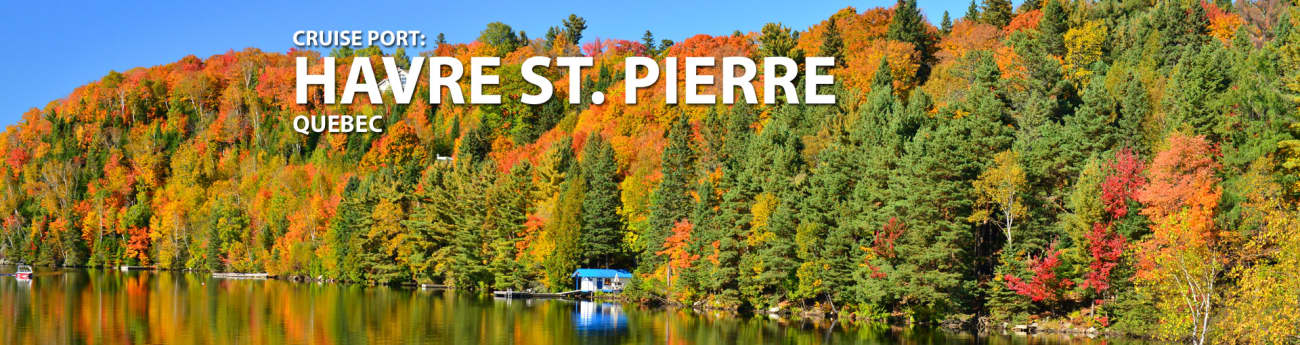This expansive autumn landscape photo, likely stitched together to create a panorama, is approximately six times wider than it is tall. Dominating the frame are tall coniferous and deciduous trees, showcasing a vibrant mix of greens, brilliant oranges, fiery reds, and bright yellows. The crisp blue sky is visible mainly in the top left corner. In the center of the scene lies a serene, mirror-like body of water — potentially a bay or lake — reflecting the stunning foliage. At the heart of the image, partially obscured by trees, stands a small white building with a blue roof, possibly a shed or shop, near a pier or wharf that extends into the water. The text "CRUZ POINT, HAVRE-SAINT-PIERRE, QUEBEC" appears in bold, white capital letters near the left-center, marking the picturesque location.